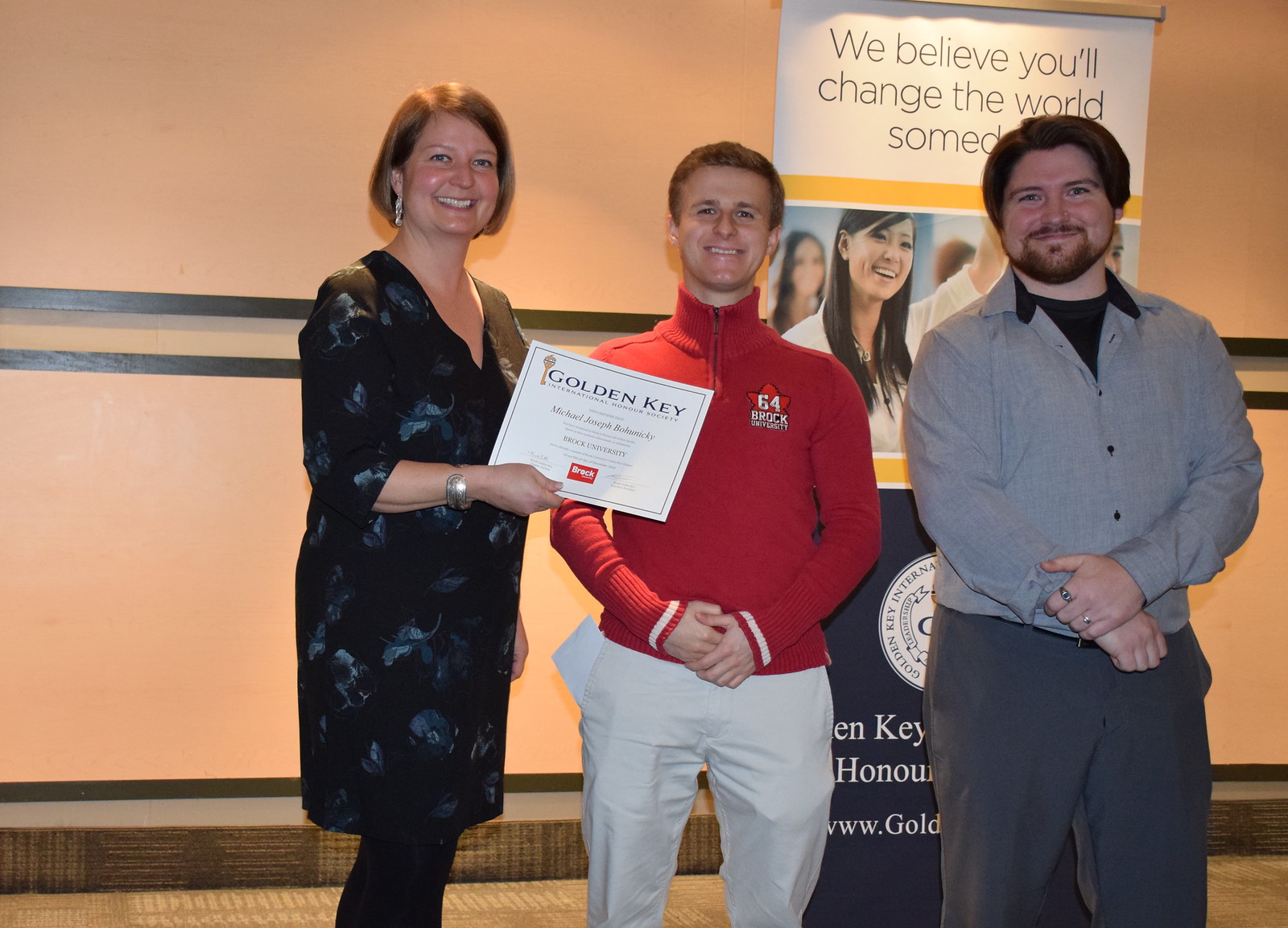In this indoor setting, the image shows three individuals standing in front of a large banner with a white wall in the background. The banner prominently displays the words, "We believe you'll change the world someday," in white and dark lettering, underscored by an image of an Asian woman raising her left hand. Below this is a segment bearing the text "Golden Key International" and an additional legible portion that reads, “Key H-O-N-O-U….”

The central focus of the image is the trio of people positioned directly in the middle. On the left is a blonde woman with short hair and earrings, wearing a blue print dress with white patches and dark stockings. She is holding an 8x6 certificate that says "Golden Key" at the top, and below that, the name "Michael Joseph Bohicke" and "Brock University." Next to her, in the center, is a smiling man with brown hair wearing a blue turtleneck jersey and white pants, his hands clasped in front of him. To his right is another man with brown hair and a mustache and beard, dressed in a gray button-up sweater over a black shirt, with gray pants. He is also smiling and has his hands clasped together in front of him.

The background features a light orange wall with horizontal dark stripes across the center and a brown border at the bottom, adding to the ambiance of the college event setting, likely associated with the Golden Key International Honour Society. The textured carpet on the ground further highlights that this is an indoor scene, possibly during an award ceremony or a similar event. The colors in the image include shades of tan, gray, brown, blue, black, red, yellow, and dark blue.